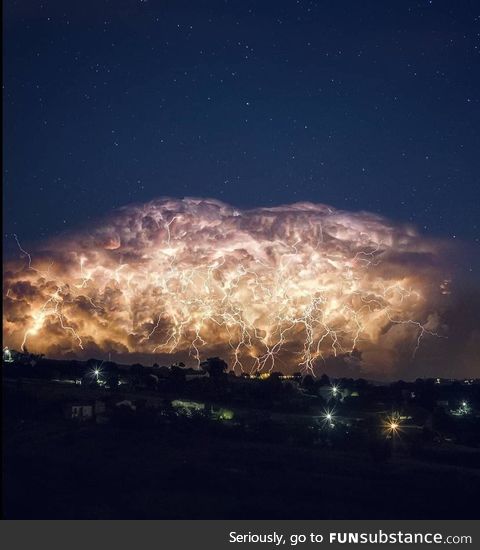The image portrays a dramatic, fantastical nighttime scene. At the top of the vertically aligned rectangular image, the sky is a deep navy blue sprinkled with tiny white stars. Dominating the center is a massive, oval-shaped cloud highly detailed in shades of gold, white, and brown, giving it a molten, lava-like appearance. This cloud is illuminated by electrifying golden lightning strikes descending towards the ground below. The cloud is so prominent it spans the entire width of the frame. Beneath this striking cloud, a dimly lit residential neighborhood is visible, with scattered lights suggesting houses amidst the darkness. At the very bottom of the image, a charcoal-colored border contains white text saying, "seriously, go to funsubstance.com," emphasizing the whimsical nature of the scene. The overall composition, rich in vibrant hues of navy, gold, brown, and occasional green and orange tones, evokes a sense of otherworldly fantasy as if capturing a cosmic thunderstorm in an imagined world.